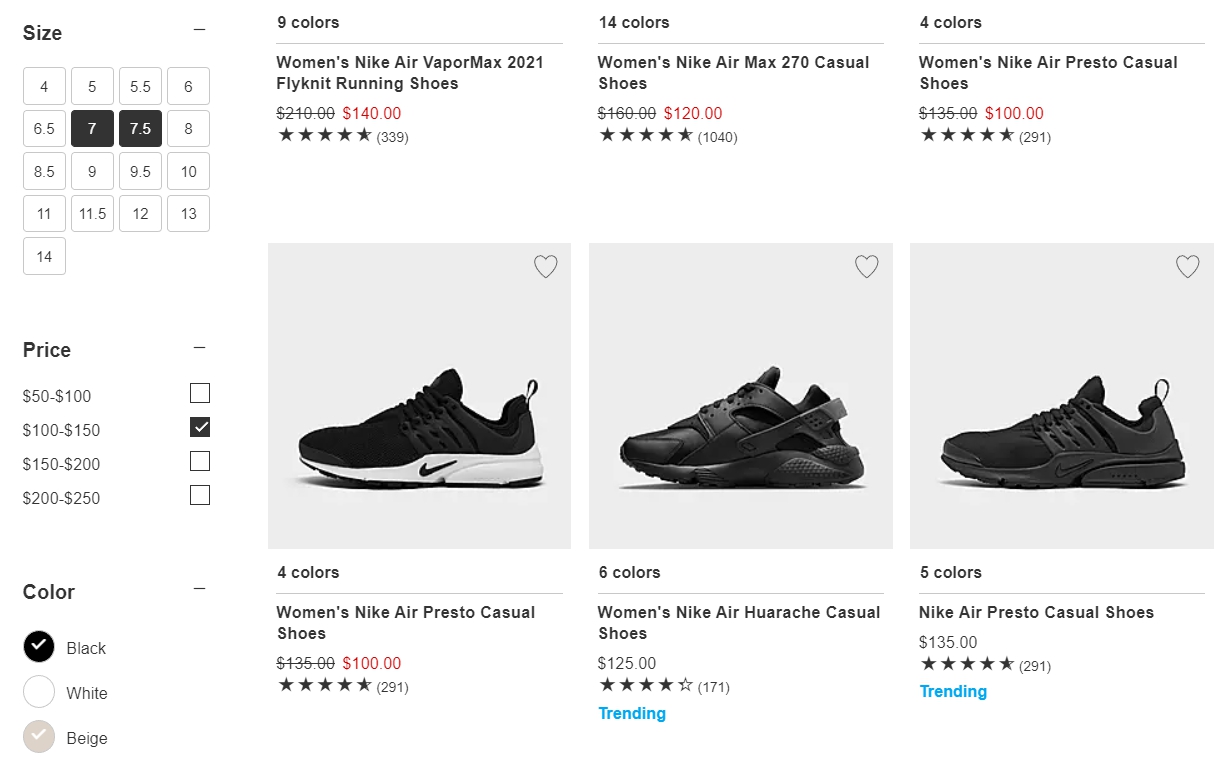The image depicts a section of the Nike.com shopping website, specifically focusing on women's footwear. Three pairs of shoes are showcased: the Air Presto, Air Huarache, and Air Presto Casual. Each shoe is displayed with an accompanying image, price, and the number of available color options. Notably, both the Air Huarache and Air Presto Casual are marked with a blue 'trending' label beneath them, indicating their popularity. On the left-hand side of the webpage, various filtering options are available, including size, price, and color, allowing users to refine their search results.